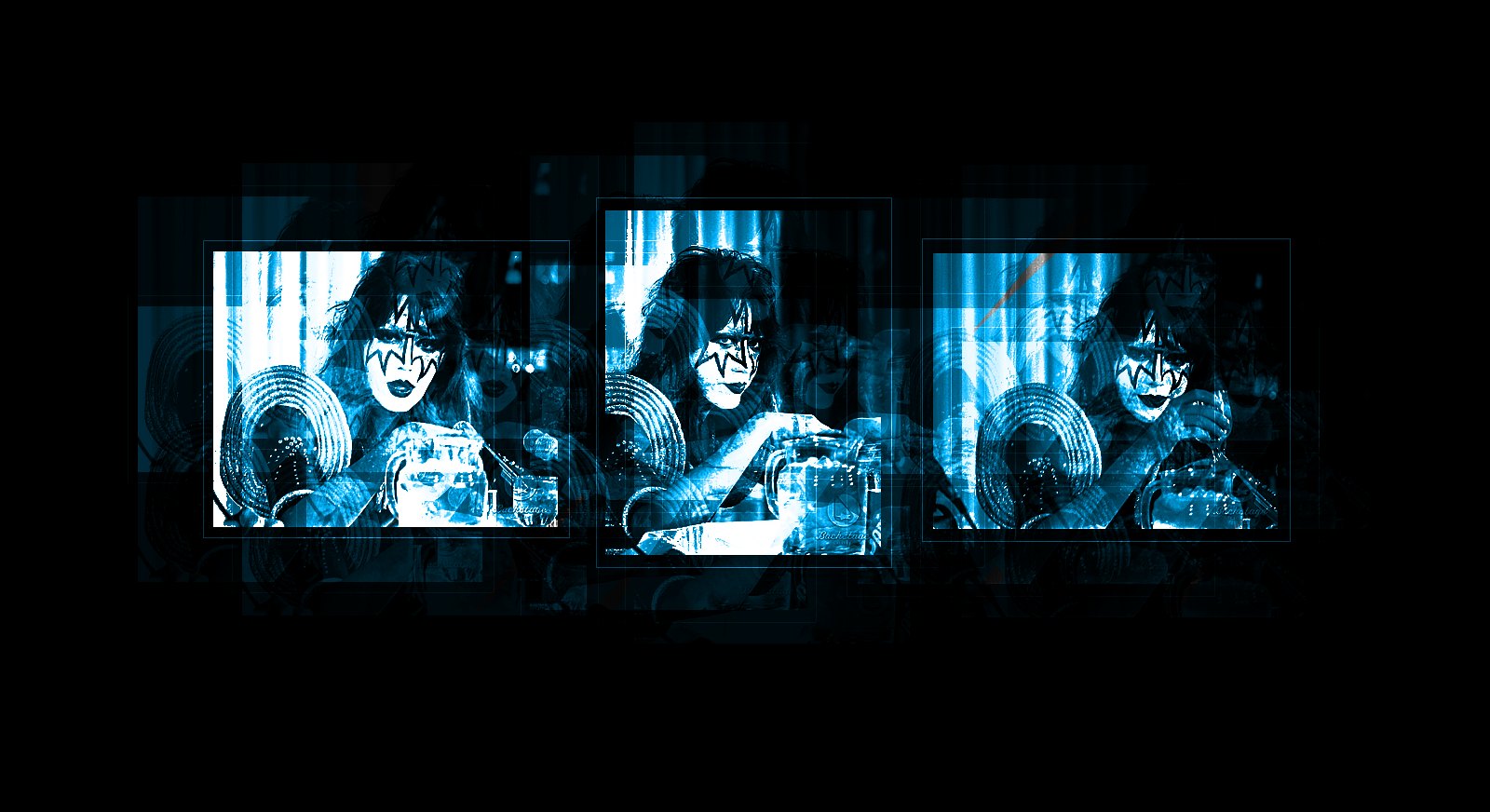In this composed image with a dark, black background, there are three distinct, bluish black-and-white photographs displayed side by side. Each shows the same member of the iconic rock band KISS, adorned in their signature stage makeup. The performer, likely Paul Stanley, is instantly recognizable with his white-painted face, long straight black hair teased at the top, and a prominent black star outline encompassing both eyes, complemented by black lipstick. 

Each image captures the musician in slightly different poses, suggesting the frames might have been taken during a single interview. The star's attire includes a leather jacket embellished with large circular silvery decorations on the shoulders. Before him on the table are a pitcher of ice water and what appears to be a microphone. The visual consistency across the photographs is punctuated by a shiny frame visible in the background of each shot. The photos, while primarily in black and white, exhibit subtle blue tints, adding a distinctive stylistic touch to the overall portrayal.